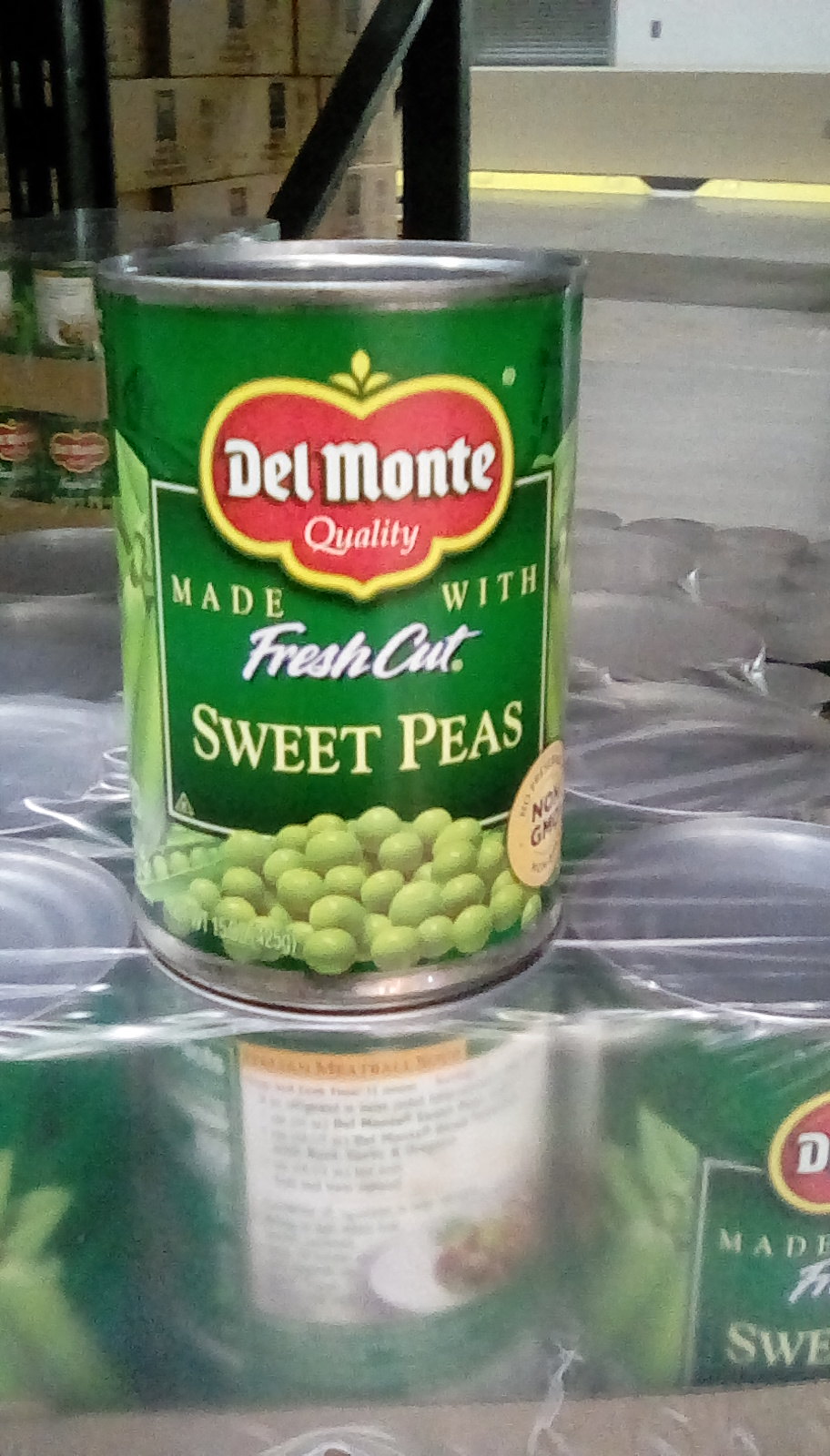This photograph captures a bustling warehouse setting with various elements composing both the foreground and background. Dominating the foreground is a plastic-wrapped package encased in a cardboard box bearing the Del Monte brand. Atop this package lies a green-labeled can of Del Monte vegetables. The can's label is detailed with a red background and white font, prominently displaying the Del Monte quality logo with a yellow ornamental design surrounding it. The label further reads "Made with Fresh-Cut Sweet Peas" in yellow and white font, accompanied by an image of green peas and a circular medallion design.

In the background, stacks of additional cardboard boxes are clearly visible, organized in towering piles. Another pallet, securely wrapped in plastic shrink-wrap, adds to the busy warehouse atmosphere. A doorway is slightly visible in the background, leading out to what seems to be a white wall with a silver item mounted on it. Sunlight streaming in casts a gentle illumination, highlighting the various textures and objects in this industrious environment.